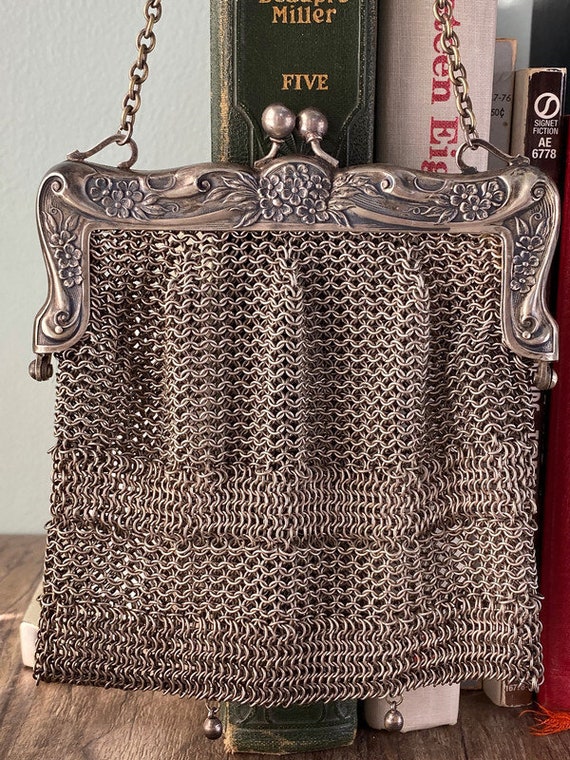This vertically rectangular, full-color photograph, likely taken using natural light, showcases a meticulously staged scene centered on a vintage chainmail purse. The purse, composed of intricate wire webbing, resembles the elegant designs from the 1930s or 1940s and has a dark aluminum coating, giving it a bronzish hue. The chainmail forms different patterns, with some links arranged horizontally and others vertically. The purse's top is adorned with a wide, ornate clasp, possibly porcelain silver, featuring delicately engraved flower designs. Two pearl-shaped knobs secure the clasp. The purse is accentuated by a small-linked brass chain attached near its edges, partially out of view. In the background, a polished wooden table supports a stack of books, one with visible "Miller 5" text. The scene is set against a neutral gray wall, creating a balanced and nostalgic composition.